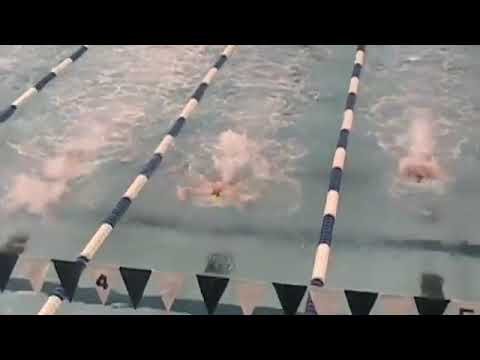This is a detailed photograph of a professional swimming pool during a race. The image captures three separate lanes, each divided by alternating blue and white ropes, with three swimmers actively competing. The water in the pool appears light blue with churned white bubbles surrounding the swimmers, indicating fast-paced movement. Overhead, a blue and white triangular banner stretches across, adorned with the numbers four and five, marking the lanes. The bottom of the pool features a dark blue stripe, and black horizontal strips frame the top and bottom of the image. This dynamic scene showcases the intensity and structure of competitive swimming.